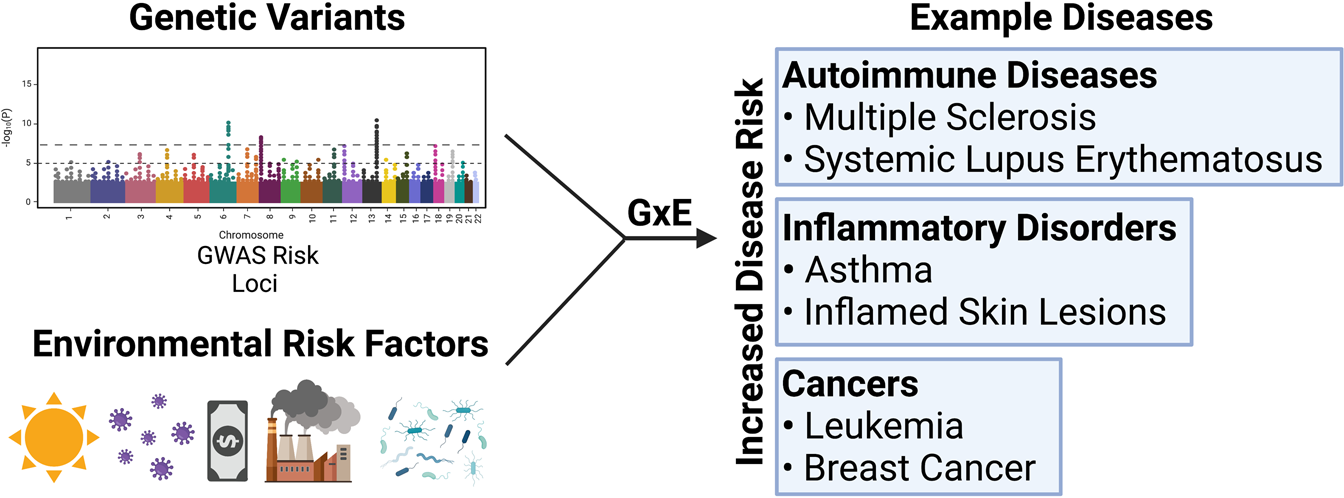This landscape-oriented color infographic illustrates the relationship between genetic and environmental factors and their contribution to disease risk. On the left side, it highlights genetic variants, labeled in black text, and environmental risk factors such as the sun, smoke from a chimney, weather patterns, pollution, germs, and even money. These are depicted through various icons. Beneath the environmental risk factors is the label "GxE" signifying gene-environment interaction, with a black triangle pointing towards the right side of the chart, indicating increased disease risk. On the right, three light blue horizontal text areas list example diseases: autoimmune diseases including multiple sclerosis and systemic lupus erythematosus; inflammatory disorders like asthma and inflamed skin lesions; and cancers such as leukemia and breast cancer. The phrase "increased disease risk" is positioned vertically along the left margin. This infographic effectively uses vivid illustrations and text to convey the interconnectedness of genetic and environmental factors in disease development.